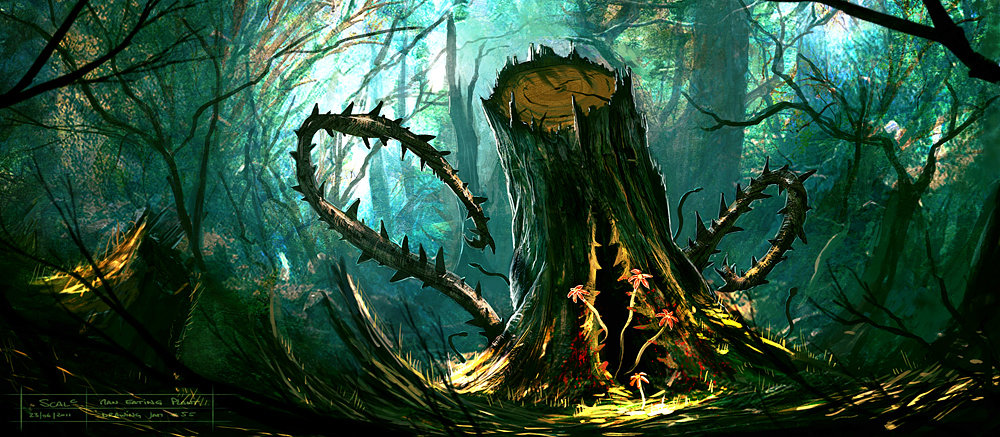This piece of digital art is a wide, panoramic illustration that seems perfectly suited for video game concept art. It portrays a dark, fantasy-themed forest with a teal-tinged sky peeking through dense trees. The central focus, slightly offset to the right, is an eerie tree stump. This stump, taller than what you'd find in a typical logging scene, is cut flat across the top and features a menacing slit down its center. This opening, skinny at the top and widening towards the base, is lined with serrated, thorny edges resembling teeth or fangs, both greenish-gold and sinister. From the base of the stump, thorny tentacle-like branches and pink-red flowers emerge, giving a sense of temptation amidst danger. The ground near the stump is dotted with what appear to be blood marks, enhancing the eerie atmosphere. The background remains shadowy and ominous, with occasional slivers of light filtering through the forest canopy, illuminating parts of the scene and adding depth to the dark, foreboding setting. Overall, the artwork exudes a captivating yet unsettling aura, drawing viewers into this creepy, fantastical woodland.